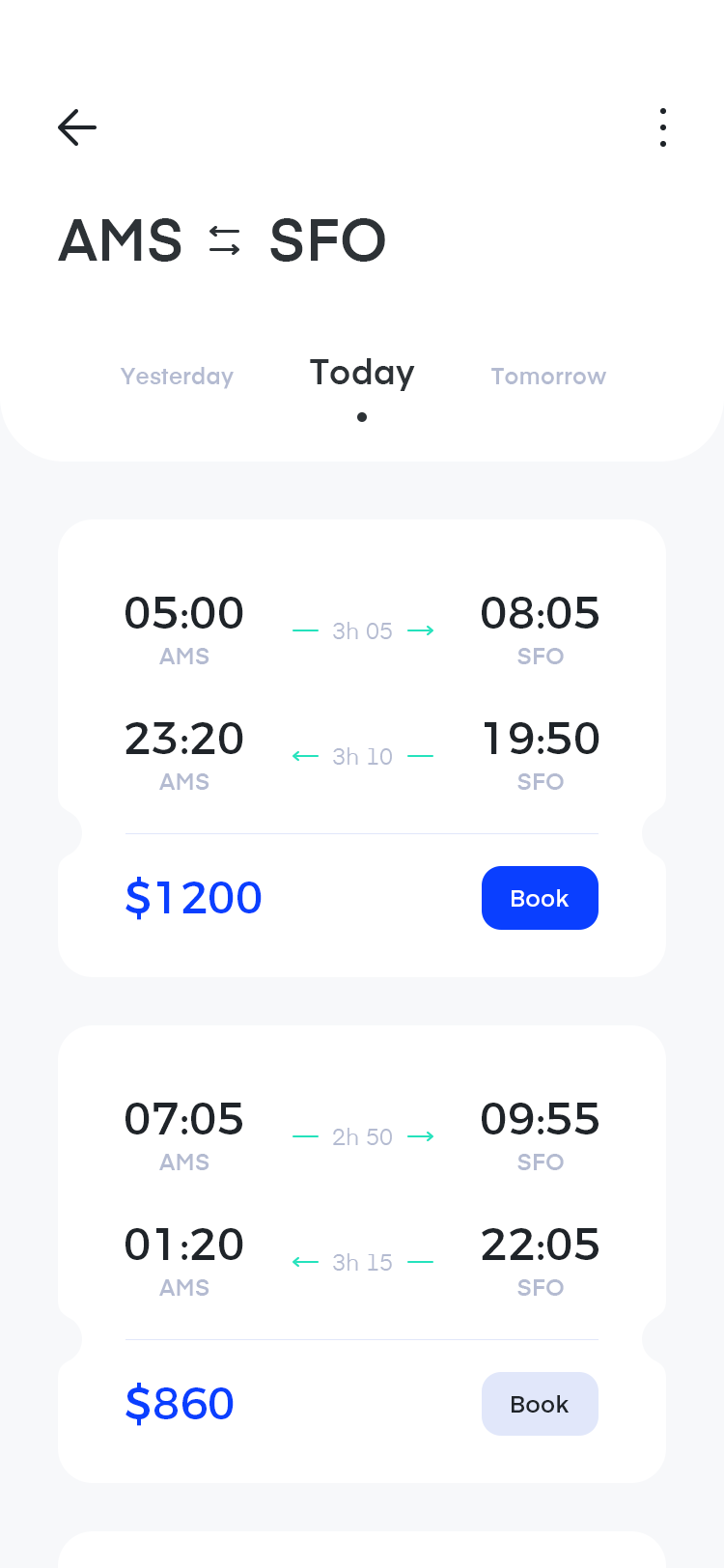This image, captured on a cell phone, displays travel information prominently at the top with the abbreviations "AMS" and "SFO" in bold black print. Arrows point between the two cities, with one arrow at the top moving from SFO to AMS and another at the bottom pointing from AMS to SFO. Below these, the words "Yesterday," "Today," and "Tomorrow" are arranged vertically with "Yesterday" appearing faint, "Today" bolded and accentuated with a dot underneath, and "Tomorrow" following similarly in line.

Further down, numbers can be seen along the left side, accompanied by arrows that point to the right and teal arrows that point back to the left, mimicking the layout above. A top rectangular section features a price of $1,200 and a "Book" button in a blue box. In the bottom left corner, another price is displayed in blue at $860, but this section lacks the "Book" option being lit up.